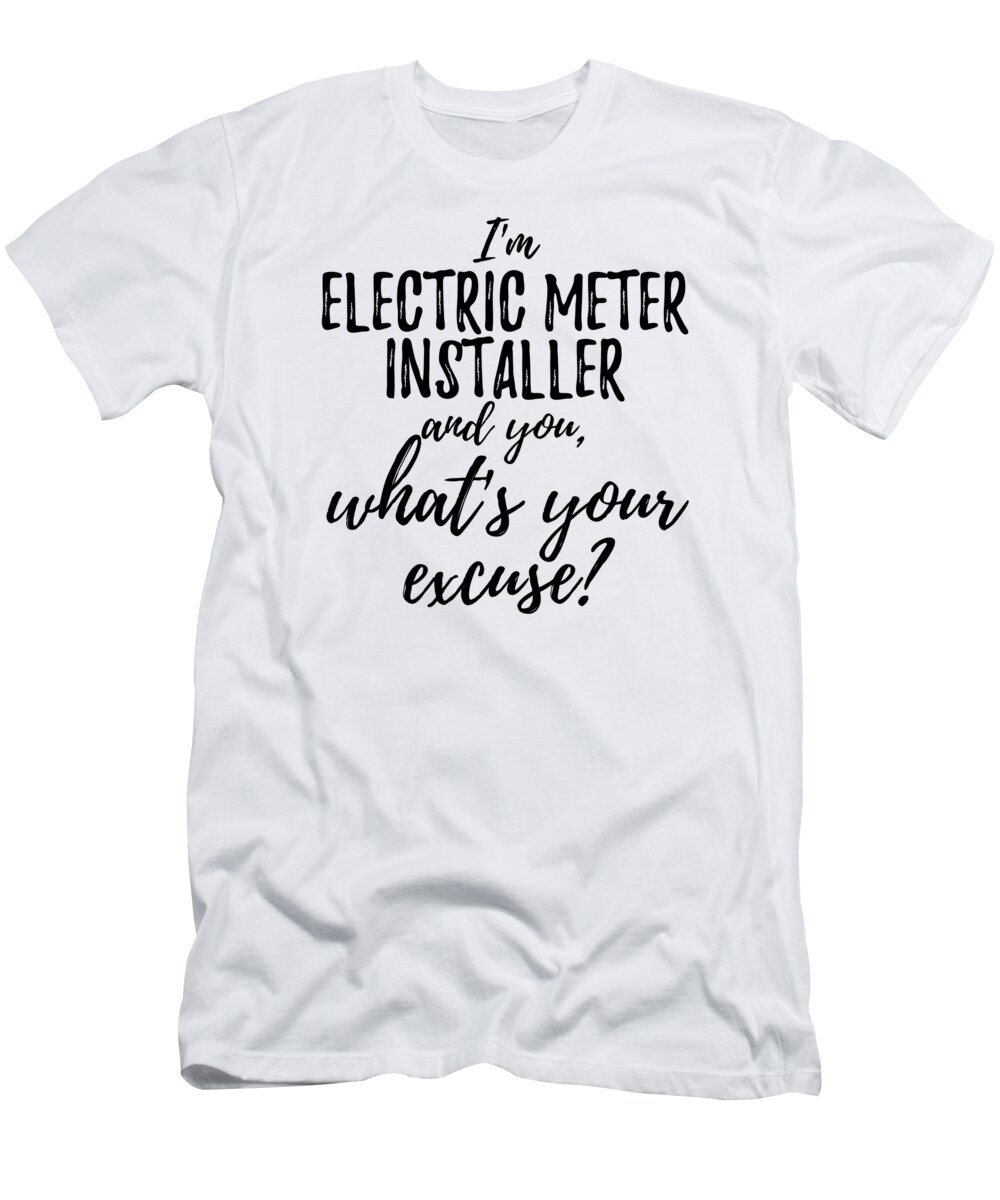This image features a white, crewneck graphic t-shirt lying flat on a white background, but it appears quite wrinkled, as if it has been balled up and neglected for some time. The t-shirt has a mixed-font inscription in black lettering. The text reads: "I'm an electric meter installer, and you, what's your excuse?" The phrase starts with "I'm" in a cursive font, proceeds with "electric meter installer" in large, block letters, and concludes with "and you, what's your excuse?" in a smaller cursive font. The text's inconsistent grammar suggests a potential translation mishap, possibly hinting at its origin from a non-English-speaking country. This quirky design seems to be aimed at those who appreciate humorous, pun-like messages on their clothing.